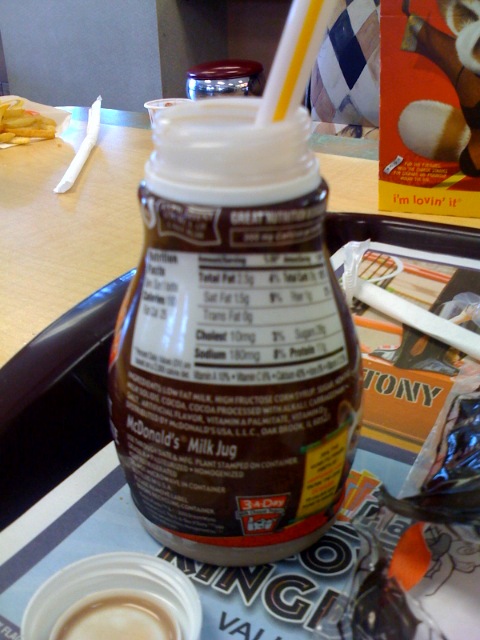A slightly out-of-focus image captures a scene at a McDonald's restaurant, focusing on a McDonald's milk jug from a children's meal prominently positioned in the center of a brown tray. The milk jug is filled with chocolate milk and showcases its white and brown nutrition label clearly. Embossed on the lower portion of the jug is the label "McDonald's milk jug." The cap, containing a small amount of chocolate milk, lies in the lower right corner of the image. Accompanying the milk jug is a yellow and white straw inserted into the milk. Scattered around the tray are two pieces of a paper straw wrapper, one at the top and another in the upper left portion. Additionally, a half-eaten container of fries is situated in the upper left section. A character resembling a brown and white animal appears in the upper right corner of the image, adding a playful touch to the scene.